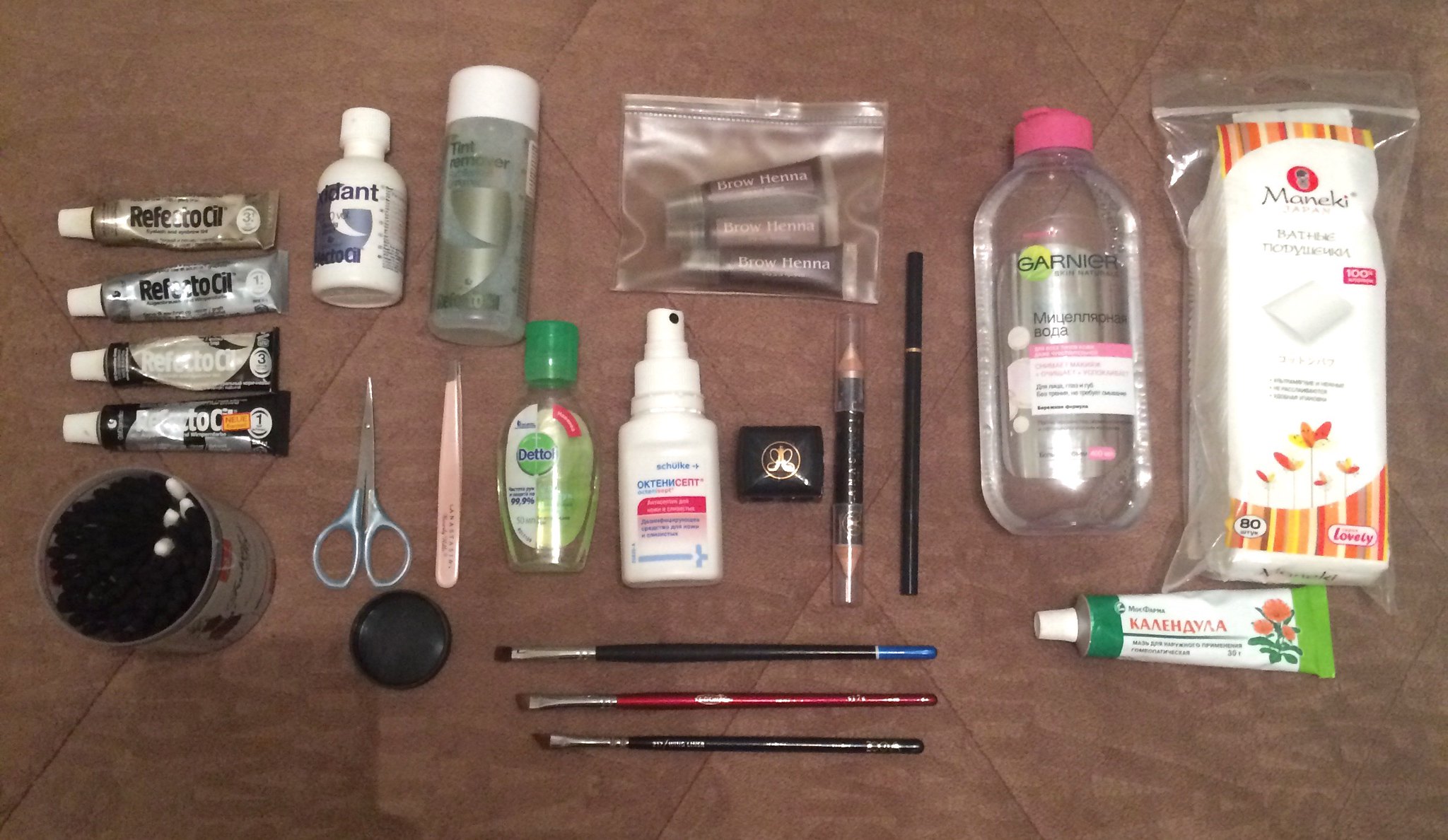The image depicts a neatly arranged collection of art supplies displayed on a brown cloth or piece of paper, captured from a top-down perspective. Starting from the left, there are several tubes of paint, each featuring varying colors and designs. The first tube is brown, followed by a silverish-white tube, another brown tube with black accents, and finally, a tube in a black casing with white caps on all of them.

Adjacent to the paint tubes is a tin cup, likely used to hold paintbrushes. Next, a white bottle with a white cap sits beside a pair of scissors. Below the scissors lies a small black cap, possibly a lid, accompanied by a round circular object. Above this is a pair of tweezers. Further up, there's a see-through, tube-shaped bottle with a white cap, containing a clear liquid.

To the right of this bottle is a plastic bag containing three small black tubes. Below this bag, there are two more bottles: one with a green cap and another white bottle equipped with a spray nozzle. Next to these bottles, there is a pencil and a pen, followed by another transparent bottle with a pink cap and clear liquid inside.

Beside this bottle rests another bag containing a piece of cloth, and below the bag lies a tube with a white cap, green top, and bottom with a white center. Finally, at the bottom of the image, three paintbrushes are neatly lined up. The detailed arrangement and variety of tools suggest an organized setup, possibly for painting or crafting.